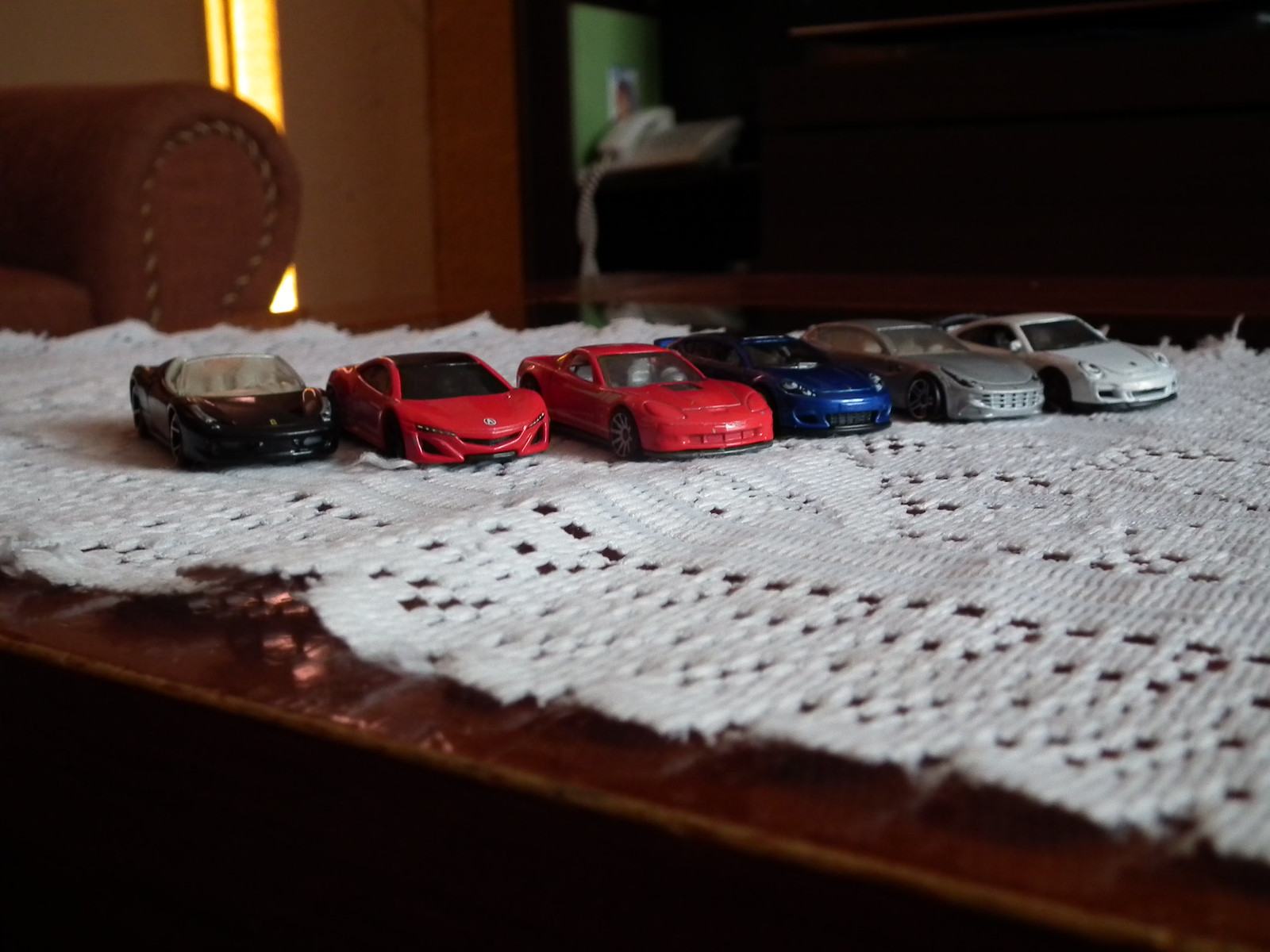In the photograph, six miniature toy cars—resembling Matchbox or Hot Wheel cars—are meticulously lined up on a white lace doily that rests atop a brown wooden table. The cars are arranged in the following order from left to right: black, red with black windows, red, blue, gray, and white. Visible in the upper left corner is the arm of a chair, distinguished by twine-colored stitching. Background details include some clutter and a telephone in the upper right, and a warm yellow light filtering in from the top left corner. Additionally, the wall in the background features a gradient of creamy to brown colors, accented by a green detail.